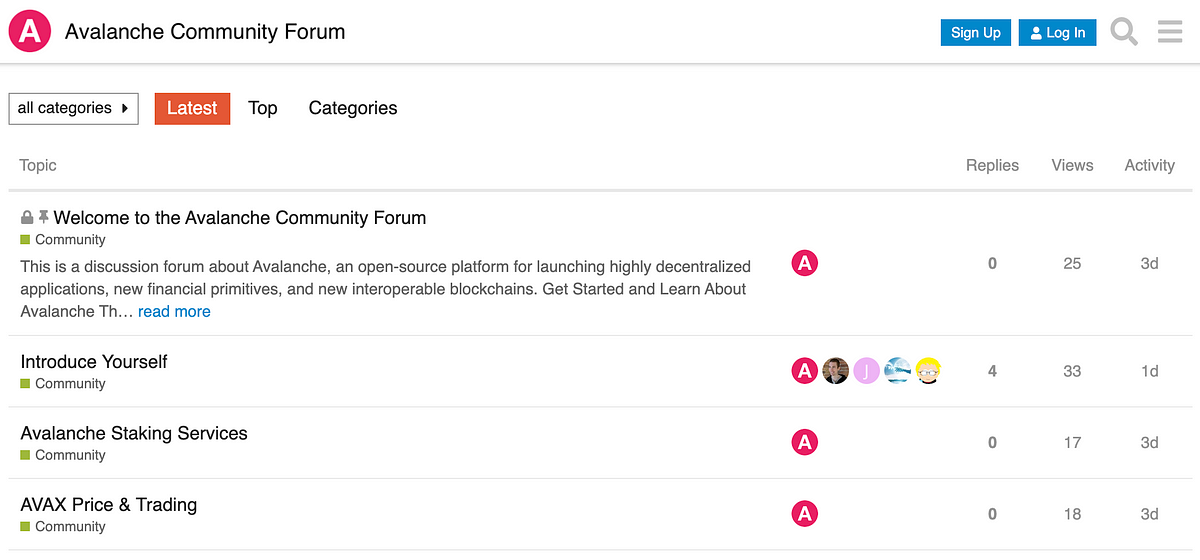This screenshot captures the Avalanche Community Forum’s homepage. The layout is set against a stark white background, with the top left corner prominently displaying the forum’s name, "Avalanche Community Forum," in bold black text. Adjacent to this, on the left, is a large pink circle featuring a white capital "A" inside it. Further right, there are two prominent blue buttons: one labeled "Sign Up" and the other "Login."

Directly underneath this header, a drop-down menu labeled "All Categories" is situated on the left, with an orange-highlighted selection for "Latest." Additional menu options include "Top" and "Categories." Below this header is where the forum content begins, structured into columns for "Topic," "Replies," "Views," and "Activity."

The first pinned post titled "Welcome to the Avalanche Community Forum" is tagged under "Community." The post introduces the forum as a hub for discussions on Avalanche—an open-source platform for launching decentralized applications, new financial primitives, and interoperable blockchains. The post encourages users to get started by learning about AverageTH and indicates that the post has zero replies, 25 views, and was last active three days ago.

Subsequent posts include:
1. "Introduce Yourself" also tagged under "Community," with four replies, 33 views, and activity from one day ago.
2. "Avalanche Staking Services and Community" showing zero replies, 17 views, and activity from three days ago.
3. "AVAX Price and Trading Community" displaying zero replies, 18 views, and activity from three days ago.